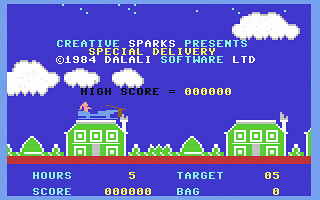This square-shaped image captures a retro gameplay screen with a light blue border, set against a darker blue background. At the top of the screen, white clouds float amidst a smattering of light blue dots, evoking a pixelated sky. The text "Creative Sparks Presents Special Delivery" is prominently displayed, suggesting the title of the game. Just beneath, there is a copyright symbol followed by "1984 Dality Software Ltd."

Further down the screen, it reads "Highscore: 000,000," indicating that either the game has just begun or no high scores have been recorded. Anchoring the lower portion of the image, a pixel art depiction features two houses, adding a touch of environmental detail to this classic gaming scene.